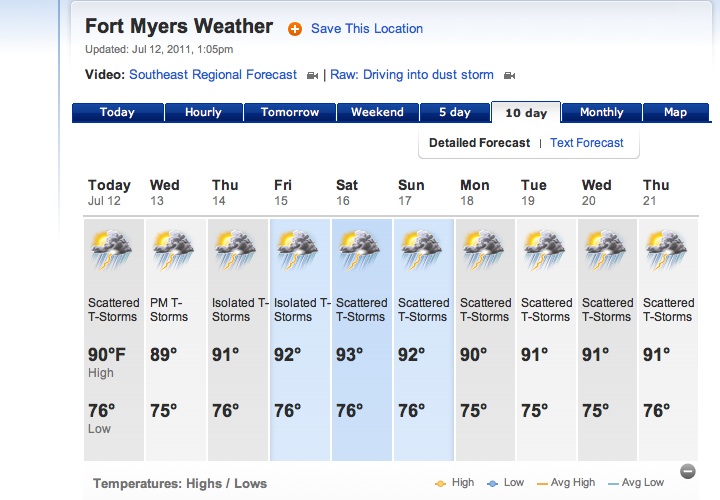**Caption:**
Fort Myers Weather Forecast (Upper Left Corner) - Dated July 12, 2011, at 1:05 PM

Save This Location (Blue, with a Red Plus Sign)

Updated Date: July 12, 2011

Video Links:
1. "Southeast Regional Forecasts" (Blue, with a Video Camera Icon)
2. "RAW: Driving Into the Dust Storm" (Blue, with a Video Camera Icon)

Forecast Navigation Options:
- Today
- Hourly
- Tomorrow
- Weekend
- 5 Day
- 10 Day (Highlighted)
- Monthly
- Map

**10-Day Detailed Forecast:**

1. **Tuesday, July 12**: Scattered Thunderstorms, High of 90°F, Low of 76°F
2. **Wednesday, July 13**: Thunderstorms, High of 89°F, Low of 75°F
3. **Thursday, July 14**: Isolated Thunderstorms, High of 91°F, Low of 76°F
4. **Friday, July 15**: Isolated Thunderstorms, High of 92°F, Low of 76°F
5. **Saturday, July 16**: Scattered Thunderstorms, High of 93°F, Low of 76°F
6. **Sunday, July 17**: Scattered Thunderstorms, High of 92°F, Low of 76°F
7. **Monday, July 18**: Scattered Thunderstorms, High of 90°F, Low of 75°F